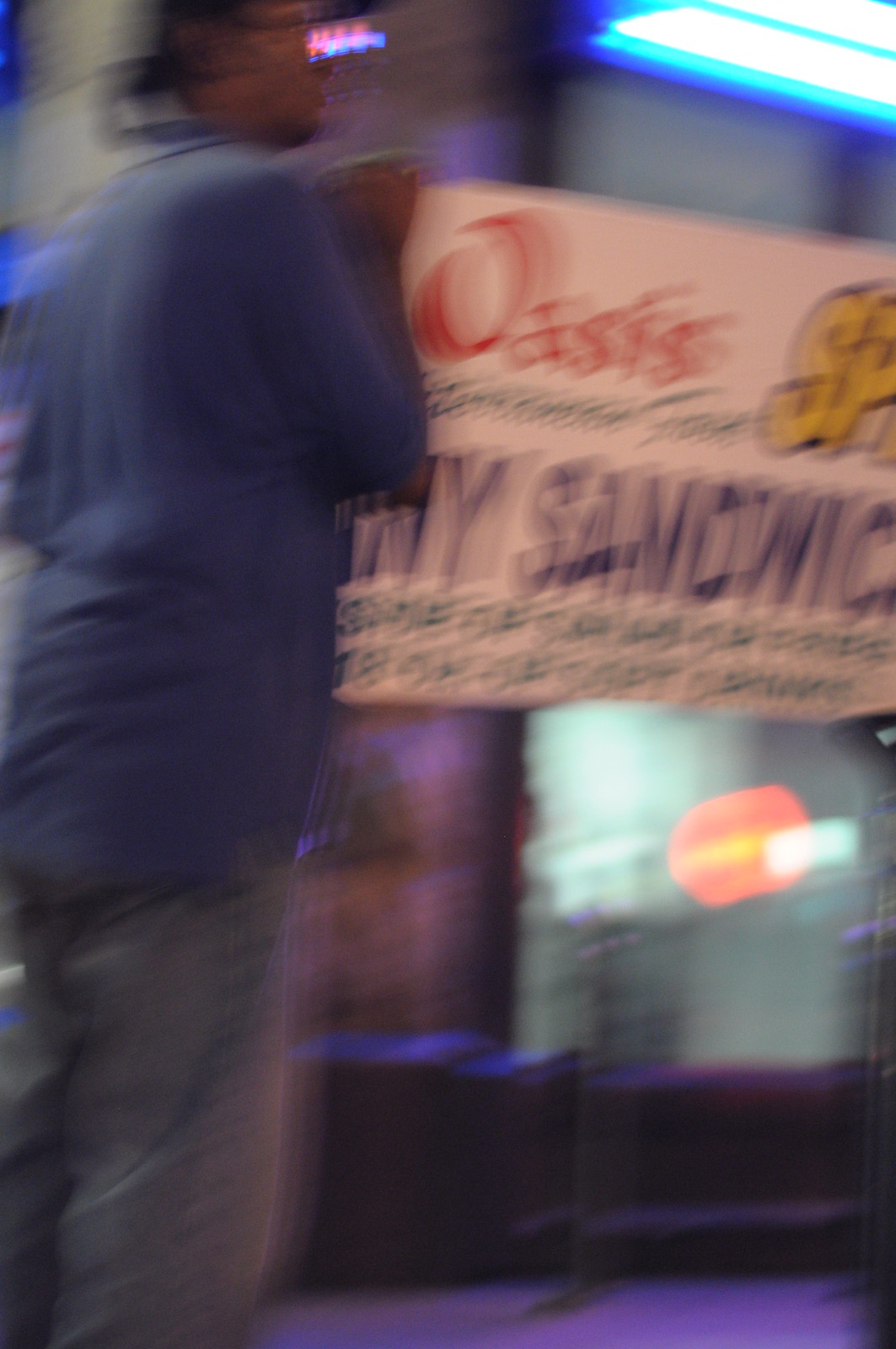In this very blurry, out-of-focus photograph taken outside at night, there's a person with medium brown skin standing on the left side, wearing a short-sleeved blue shirt and gray pants. They appear to be contemplating a hand-painted, wooden sign that dominates the right side of the image. The sign, mounted above a purple-colored wall with a glass window, is illuminated by a blue fluorescent light in the upper right corner. Above the window, the sign displays the words "Oasis, NY Sandwich" with the letters in red, yellow, and blue, though some letters are missing or obscured by blurriness. Concrete is visible below the window, adding to the scene's gritty, quirky atmosphere. The overall effect of the photograph, with its combination of blurred lights and indistinct details, leaves an enigmatic, almost otherworldly impression.